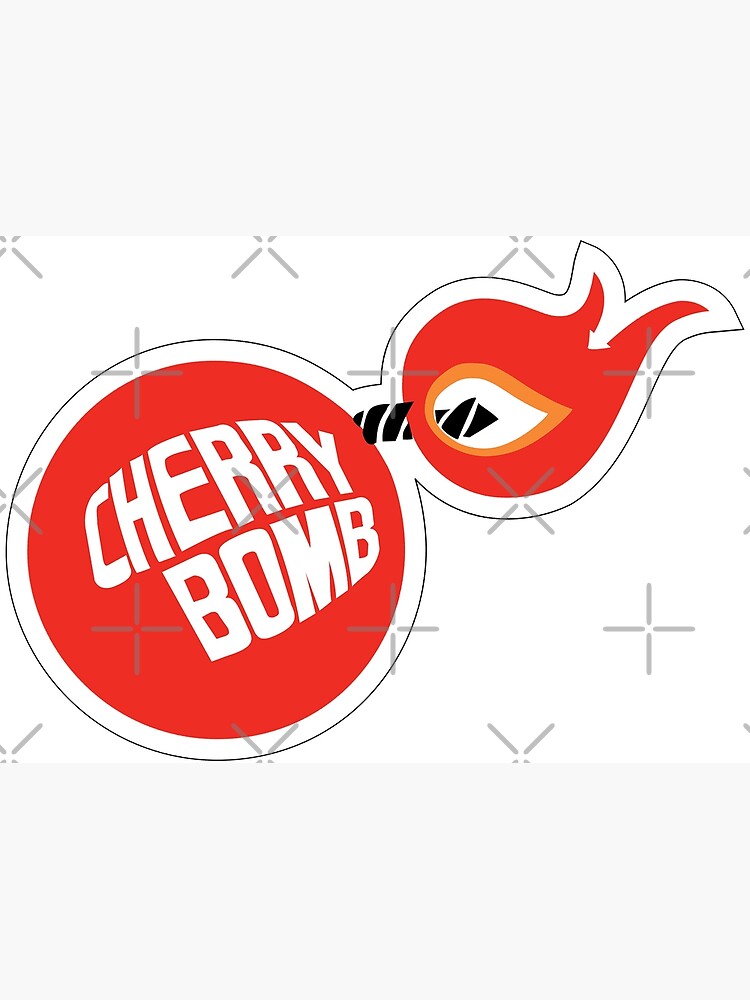This detailed graphic illustration features a central red circle prominently labeled "CHERRY BOMB" in large, distorted white letters, creating a fisheye effect to mimic the curvature of a spherical object. The graphic is reminiscent of a classic cherry bomb, an explosive device historically known for its loud bang. Emerging from the upper right side of the circle is a black-striped wick, cartoon-style, which appears freshly lit, as evidenced by an eye-catching flame. This flame, intricately drawn, features a bright red outer glow, a slightly darker orange inner core, and a transparent white center that reveals the wick underneath. The flame's red portion forks at its end and forms an inward-pointing arrow. The entire image is set against a white background, flanked by very light gray banners or borders at the top and bottom, framing the central graphic. There is also a black outline enclosing the red circle, giving it a sticker-like appearance. The image includes distinguishable X's and check marks as watermarks on the front, suggesting it is intended for purchase, perhaps for use in newsletters or advertisements.